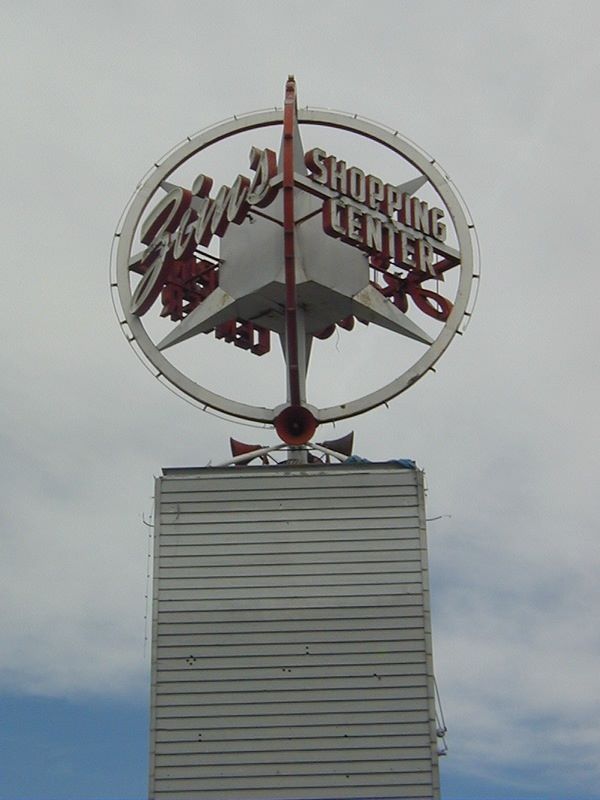The image features a high-resolution photograph of the uppermost portion of a building. Prominently, there is a 3D sign or antenna-like projection emerging from the rooftop. The sign is circular, divided into two sections. The left half displays the word "ZIMS" in a cursive font, while the right half reads "Shopping Center." Central to the circle and behind the text is a star-shaped design. This unique structure rests atop a rectangular section of the building, all rendered in a soft, light gray hue. The backdrop of the scene is a cloudy sky, adding an atmospheric touch to the composition.